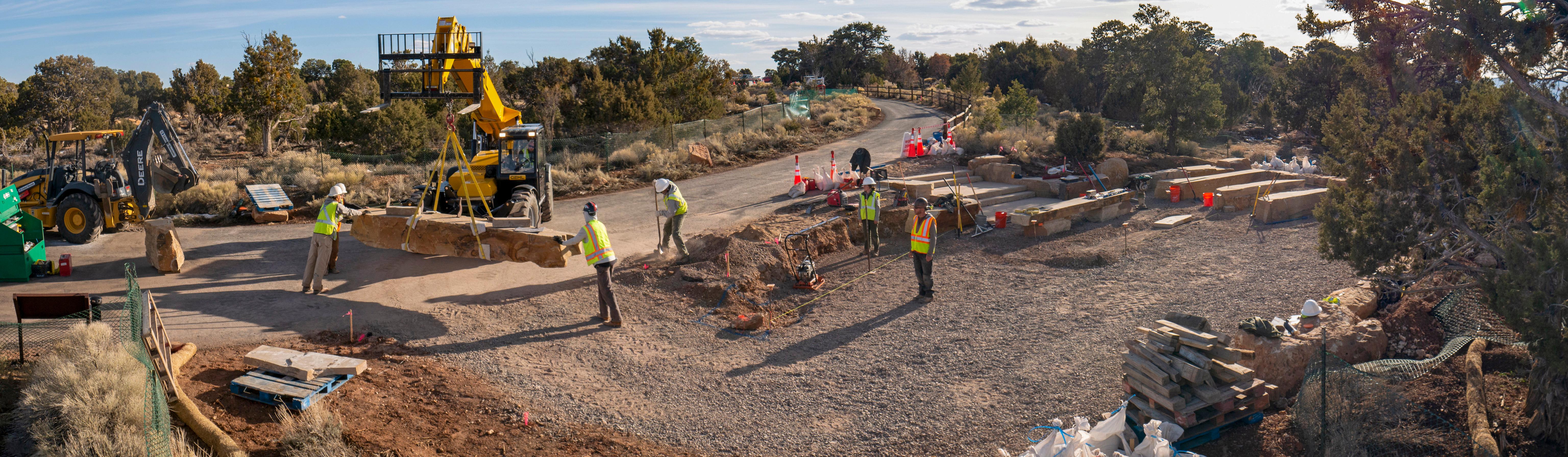The image depicts a bustling construction site featuring a variety of equipment and workers. At the center is a prominent yellow and black forklift carrying a large piece of timber secured with yellow straps. Construction workers in neon yellow vests are strategically positioned around the forklift, actively guiding its operation. To the left of the forklift, a yellow and black backhoe stands idle. The ground, covered in gravel and gray rocks, also includes a concrete path leading through the site.

A staging area is visible with several long, rectangular boxes seemingly prepped for integration into the ongoing construction work. Scattered around this area are bright orange cones and buckets.

In the background, a fence marks the boundary of a forested area with low trees and extensive light brown grass, suggesting a drought-affected environment. Overhead, the sky is a clear blue with a few low white clouds. The image captures the coordination and activity typical of a dynamic construction site set against a natural backdrop.